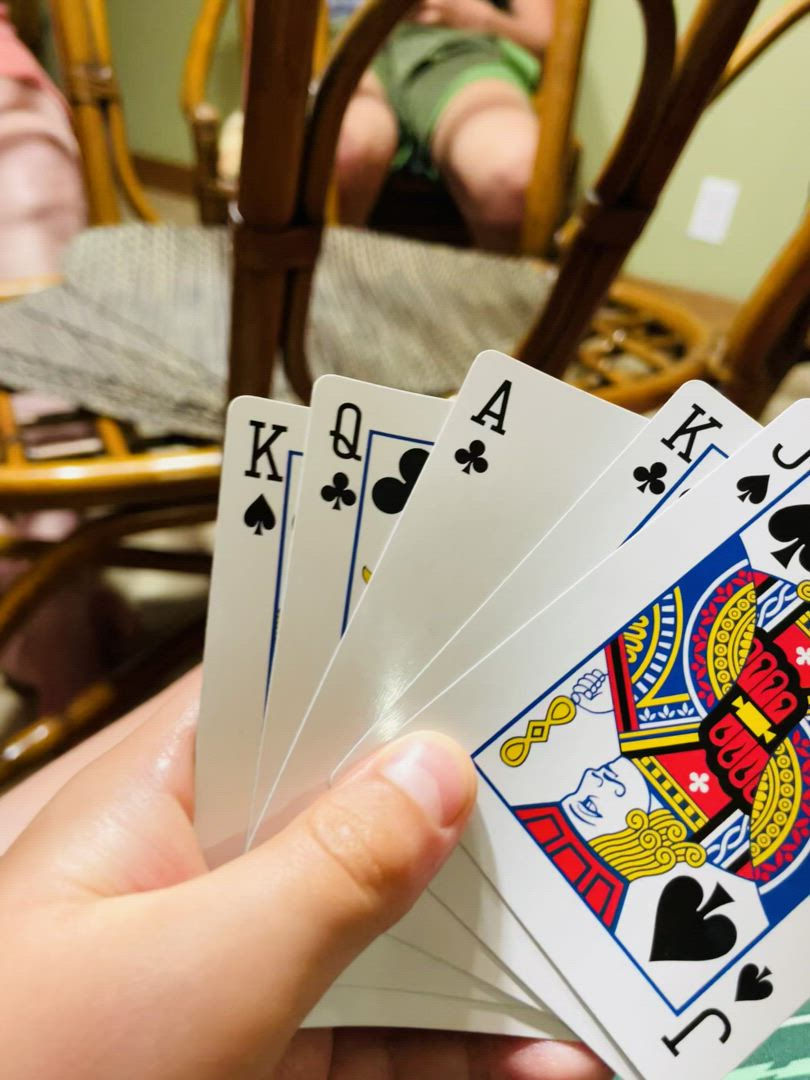In this close-up shot, a hand holds a set of playing cards, prominently featuring the King of Spades, Queen of Clubs, Ace of Clubs, King of Clubs, and Jack of Spades. The cards are fanned out, with the Jack positioned at the bottom right. The background reveals a kitchen table setting, blurred to maintain focus on the cards. Seated around the table are a few people, with only one person clearly visible at the back left side. The walls are painted an olive green, and a white power socket can be seen on the right side of the image. The overall ambiance is that of a casual game night in a warmly lit kitchen.